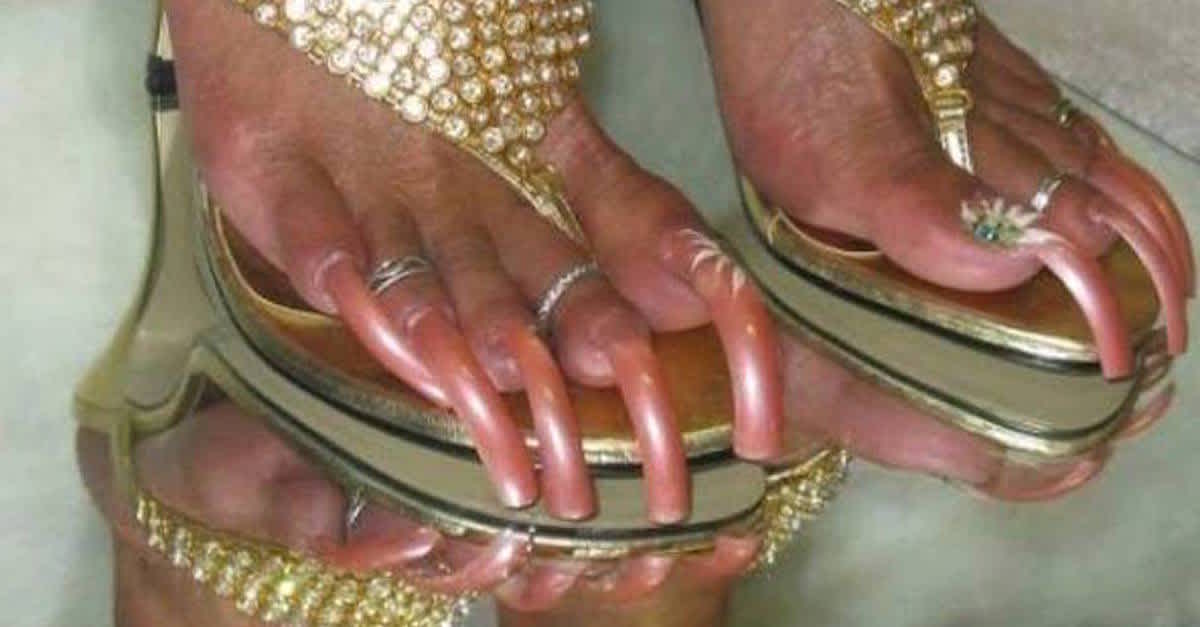The image depicts a pair of feet, likely belonging to a woman, adorned with extraordinarily long, curved toenails that extend up to about two to three inches. The toenails are painted a pale orange or pink and one nail features an intricate white flower-like design, complete with petals. The second and fourth toes on one foot are decorated with silver rings. The woman is wearing elaborate, gold thong-like sandals embellished with crystals and spangles. The sandals have extremely high soles to accommodate the lengthy toenails and rest on a glass or mirror-like surface that reflects the feet and nails. The image appears to be captured indoors, possibly in a setting like a nail salon.